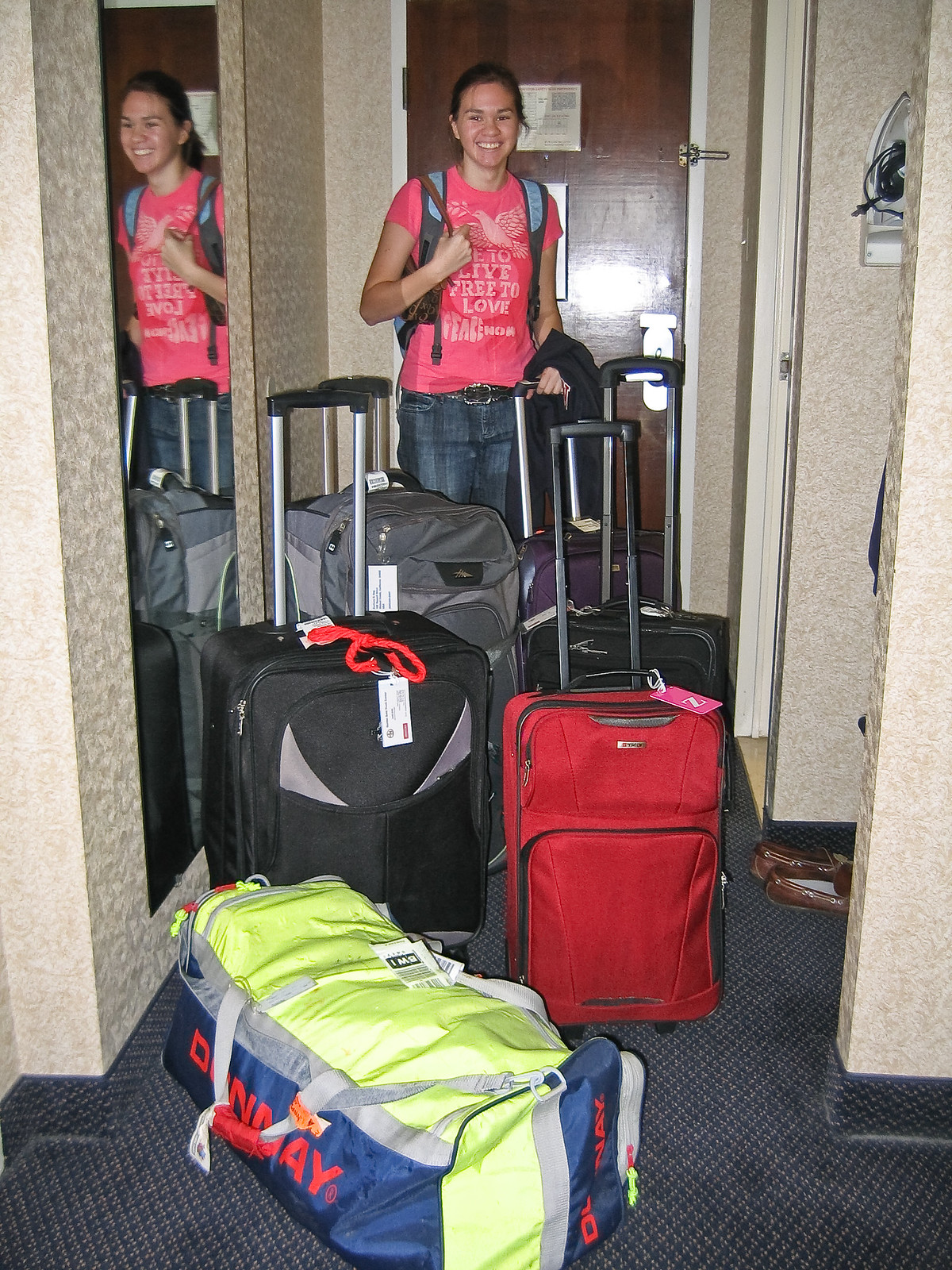In this photograph, taken inside a hotel room, a young woman stands smiling in front of a chocolate brown hotel door with a metal latch. She appears to be in high school, wearing a pink shirt that says, “to live free to love, peace now,” partially obscured by her hand. She has her hair tied back in a ponytail and is dressed in blue jeans with a black belt and brown boat shoes to her right. A black backpack with blue inserts and a small purse are draped over her shoulders, while a jacket hangs over one arm.

In front of her are five suitcases and a duffel bag, all with their handles pulled up as if she is ready to leave. She stands holding a purple suitcase. Directly in front of her are a black and a red suitcase, both with luggage tags. Behind these are two more suitcases, one gray and one black. The blue duffel bag in front features red writing and airport tags. The brown shoes are on the darkish blue and tan-patterned carpeted floor. The walls behind her have a busy textured beige pattern, with a hotel iron affixed to the wall on the right and a mirror to the left reflecting her and the luggage.